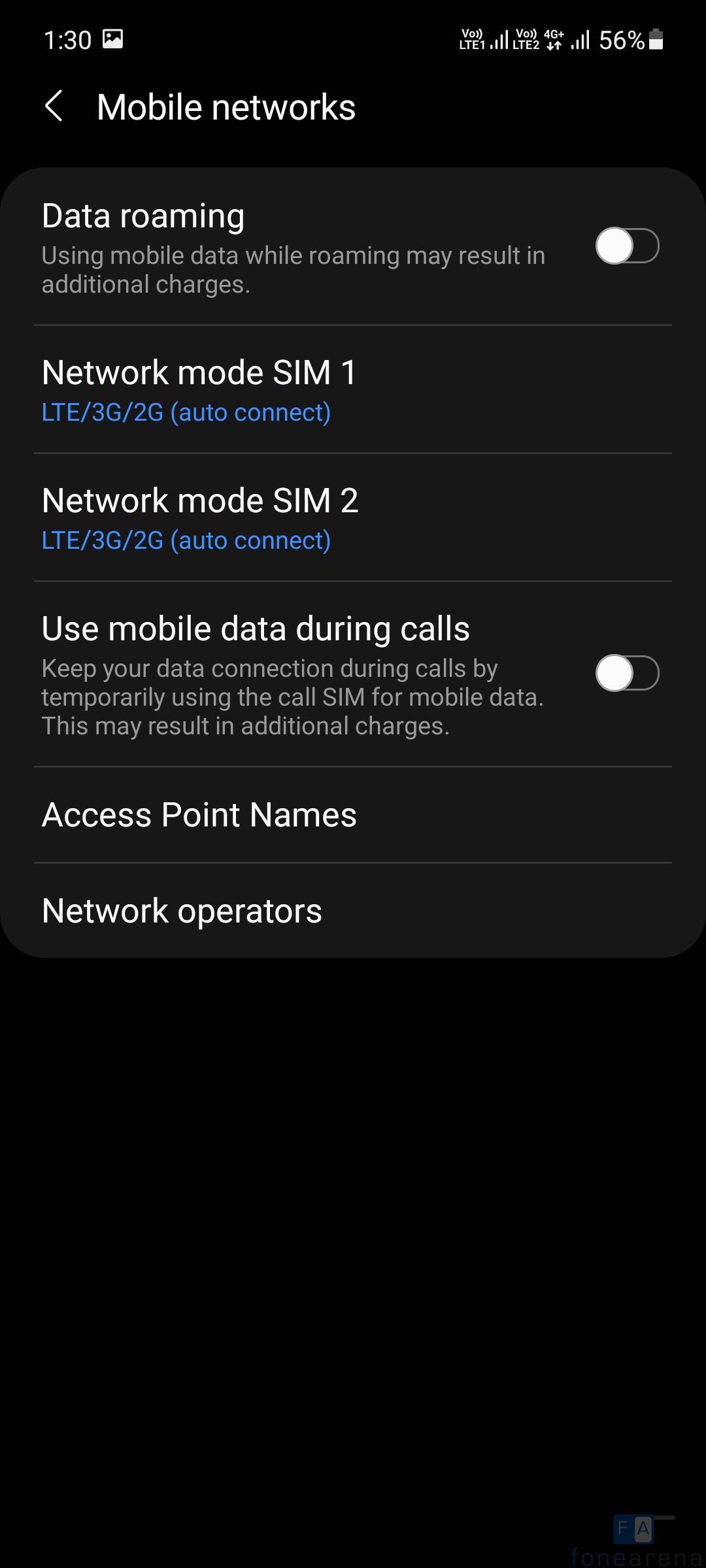A detailed screenshot of a mobile device's network settings page captured against a black background with predominantly white text and selective blue highlights. The time displayed in the upper left corner is 1:30. Below the time, the primary heading reads "Mobile Networks" in white. The first option listed is "Data Roaming" accompanied by a succinct description and a faint white slider button to the right.

Following this, the "Network Mode SIM 1" entry is detailed in white text, with the selected mode "LTE/3G/2G Auto Connect" highlighted in blue. Adjacent to this, under "Network Mode SIM 2," the same description and blue-highlighted mode configuration are displayed, indicating "LTE/3G/2G Auto Connect."

A faint white line separates these sections from the next setting, "Use Mobile Data During Calls," which includes a white slider button and a description aimed at keeping the data connection active during calls. Further down the page, the "Access Point Names" and "Network Operators" options are listed in white text. The lower portion of the screen reveals a blank area set against the black background, completing the interface's simple yet functional aesthetic.